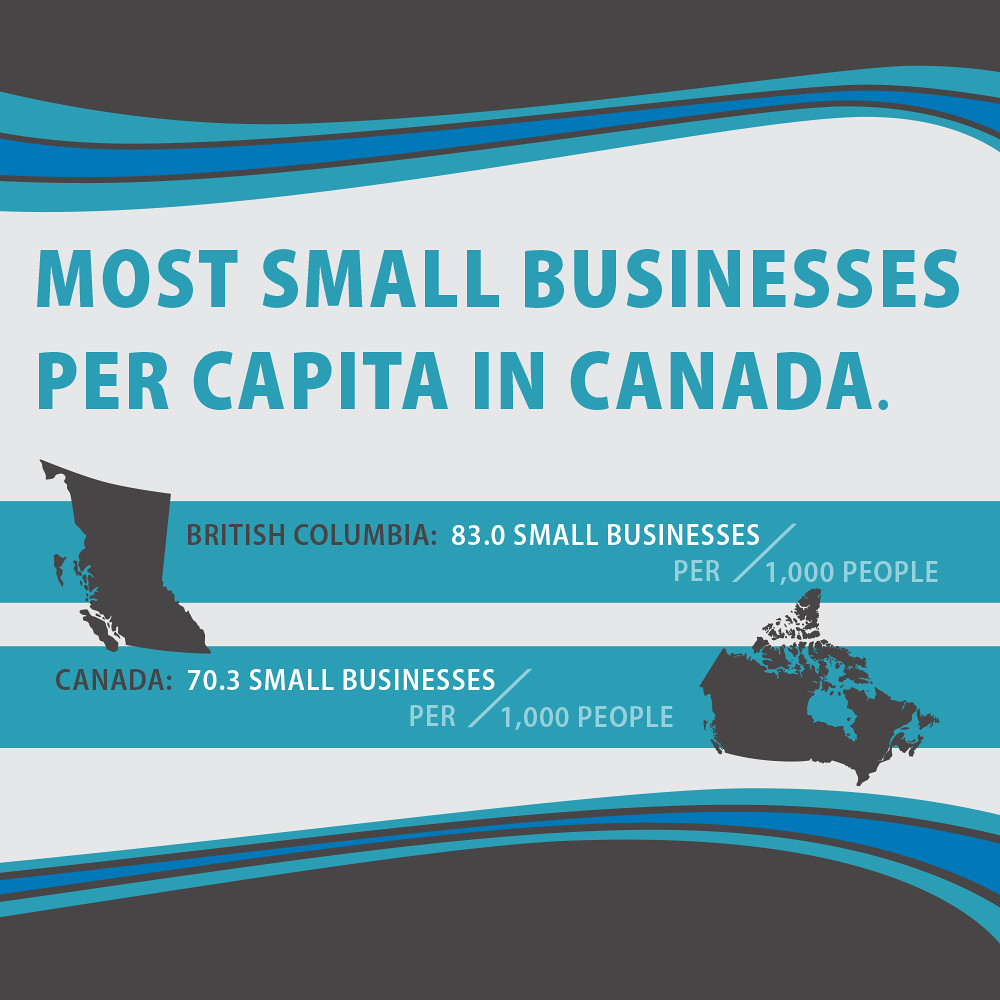The image is an infographic poster titled "Most Small Businesses Per Capita in Canada" in bold turquoise block lettering, approximately two-thirds of the way up from the bottom. The background features a central white area flanked by black sections at the top and bottom, and wavy spiral patterns in dark blue and light blue.

Centered on the poster, two turquoise horizontal bars highlight key data. The first bar features a black silhouette of British Columbia on the left, with the label "British Columbia:" in black text to the right, followed by "83.0 Small Businesses per 1,000 people" in white text. Below, a second turquoise bar presents a black silhouette of Canada, labeled "Canada:" in black text, with "70.3 Small Businesses per 1,000 people" in white text.

The layout and color scheme uses a mixture of dark, greyish blue, and turquoise hues, drawing attention to the comparison of small business densities between British Columbia and the entire country of Canada.